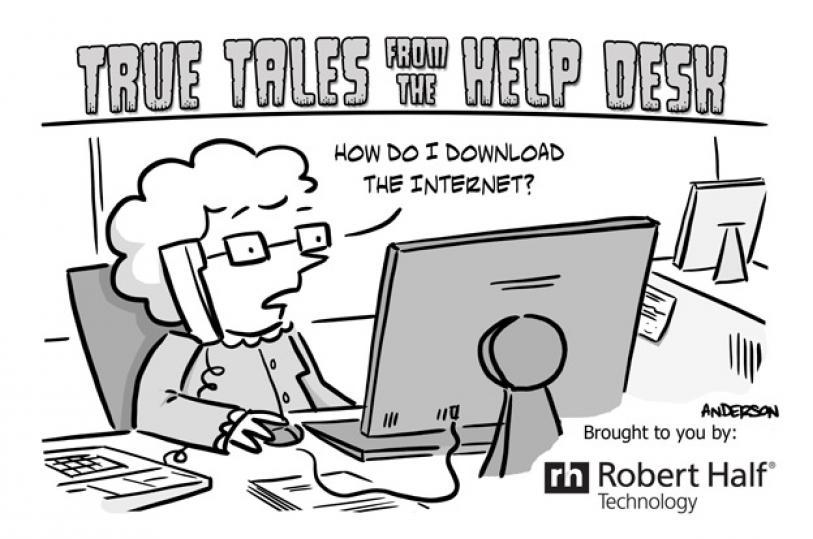This black, white, and gray comic panel titled "True Tales from the Help Desk" features an elderly woman with short, curly hair and square glasses. At the top, the title is presented in gray letters with a black outline and underlined in black. The woman, seated in an office environment, is holding a computer mouse in her right hand while balancing a corded telephone on her shoulder. With her mouth open wide, she puzzledly asks, "How do I download the internet?" in a speech bubble. The cartoon humorously illustrates the kind of naive inquiries often encountered by help desk workers. At the bottom right, the panel credits "Anderson" and is marked with the phrase "Brought to you by Robert Half Technology," accompanied by the RH logo inside a square.